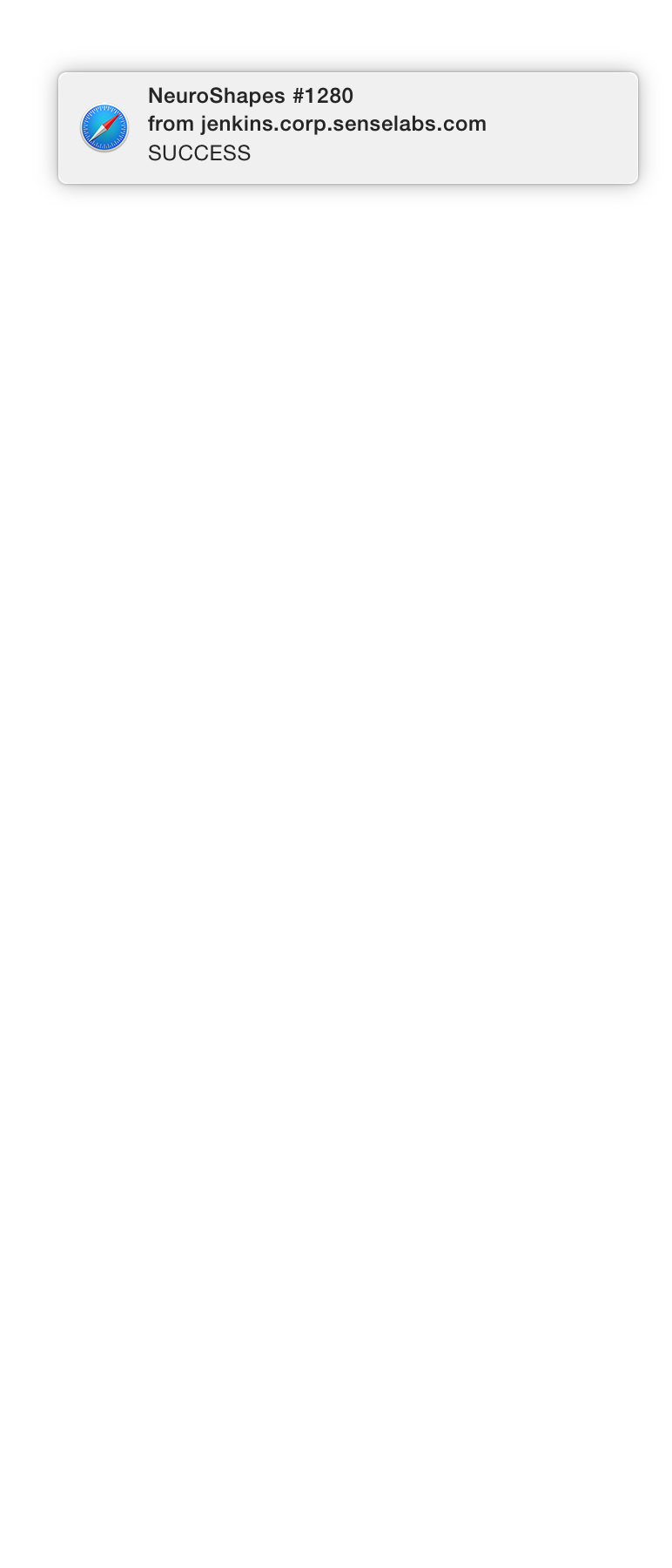The image is a large, vertical white rectangle with minimal content. Centered within this vast white space is a small horizontal gray rectangle. Inside this smaller rectangle is black text that reads: "Neuro Shapes Number 1280 from Jenkins (J-E-N-K-I-N-S) dot corp (C-O-R-P) dot SenseLabs (S-E-N-S-E-L-A-B-S) dot com." Below this text, the single word "Success" is written. 

To the right of the text is a blue compass icon with a red and white needle. The compass face is adorned with light gray dashes instead of numbers.

The overall color scheme consists of blue, gray, red, white, and black elements against a predominantly white background, emphasizing the sparse but specific information presented within the image.